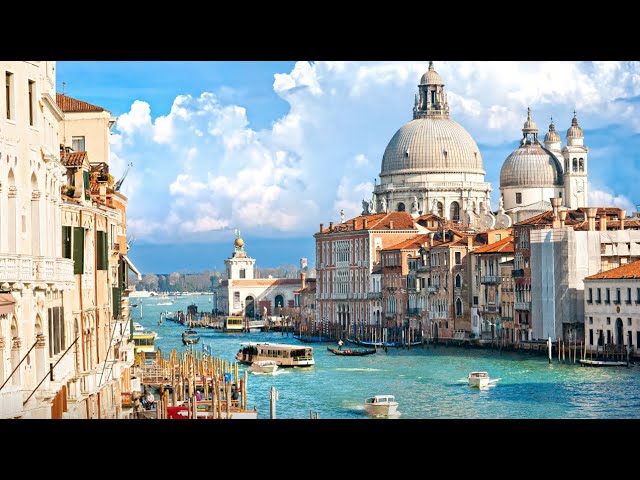This captivating image portrays a vibrant canal scene in what appears to be Venice, Italy. The wide, greenish-blue canal is bustling with activity, featuring a variety of boats including ferry boats, motorboats, gondolas, and small personal vessels. On both sides of the canal, three to four-story buildings, adorned with clay and red brick roofs, line the waterway, exuding an old-world European charm. Some buildings are designed with intricate domes and turrets, while others have a more traditional Italian architecture, with beige and white facades. 

On the right side of the canal, a majestic church with two large cathedral-style domes and a smaller dome or balcony stands prominently in the background. In the foreground, small piers and pylons can be seen, along with columns topped with crosses. The sky above is a magnificent blue, adorned with big, puffy white clouds, illuminated by the sunlight, adding to the picturesque and sunny ambiance of the scene. The distant horizon reveals a hint of greenery, possibly indicating trees not directly on the water. This image is horizontally rectangular and framed with black bars at the top and bottom, emphasizing the scenic beauty captured within.